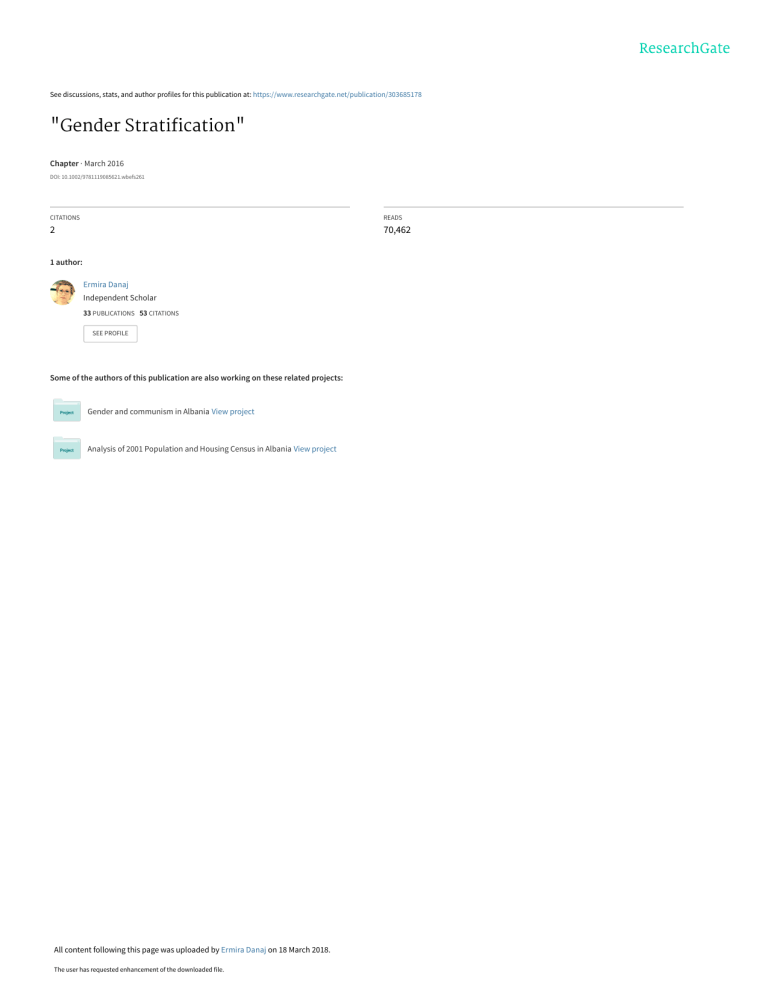This image depicts a webpage from Research Skate showcasing details of a publication. The webpage displays information about a publication titled "Gender Stratification." The text is highly blurry, but zooming in reveals the following: "See discussion stats and author profiles as far as publication." The publication can be found at https://www.researchskate.net/publication/30365178 and is from March 2016, cited 2 times and read by 70,462 individuals.

One author, Amira Dhanaj, an independent scholar, is featured prominently. Amira has 33 publications and 53 citations to their name. The profile provides insights into Amira's academic contributions, and mentions that they are currently working on related projects, specifically: "Gender and Communism in Albania" and "Analysis of 2001 Population Census in Albania." The page includes links for further exploration of these projects, highlighting Amira's engagement in comprehensive research on gender and demographic issues in Albania.